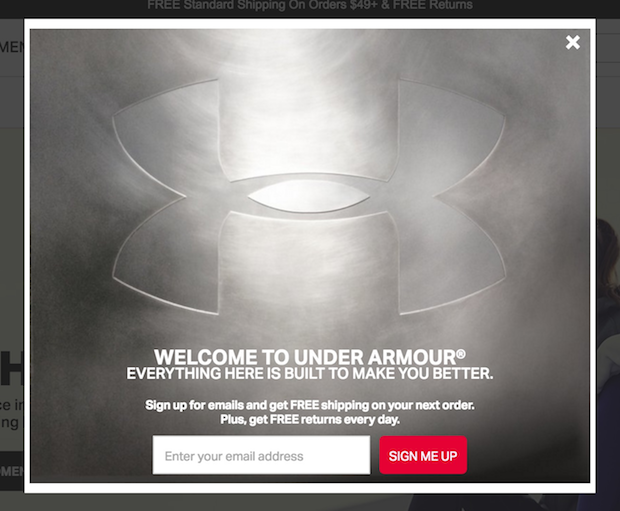This is a detailed descriptive caption for an image of a sign-up pop-up for Under Armour on an e-commerce site. The background of the image showcases various photographs, albeit grayed out to draw attention to the pop-up. The pop-up itself promises enticing benefits: free standard shipping on orders of $49 and above, along with free returns.

The pop-up features a prominent Under Armour logo, where the iconic "UA" is visually intersected and appears stamped into a realistic, textured aluminum surface, showcasing specular highlights that enhance its metallic look. Within a white border, bold all-caps text welcomes visitors with "WELCOME TO UNDER ARMOUR" and the message "EVERYTHING IS BUILT TO MAKE YOU BETTER". 

Below the welcome message, users are invited to sign up for emails with the incentive of free shipping on their next order and free returns every day, both benefits highlighted in all caps. The user is prompted to enter their email address in a white input field accompanied by a pink button with white text reading "SIGN ME UP". For those not interested, a small white "X" in the upper right corner allows them to close the pop-up. This strategic pop-up aims to build their mailing list by offering practical perks in exchange for an email address.